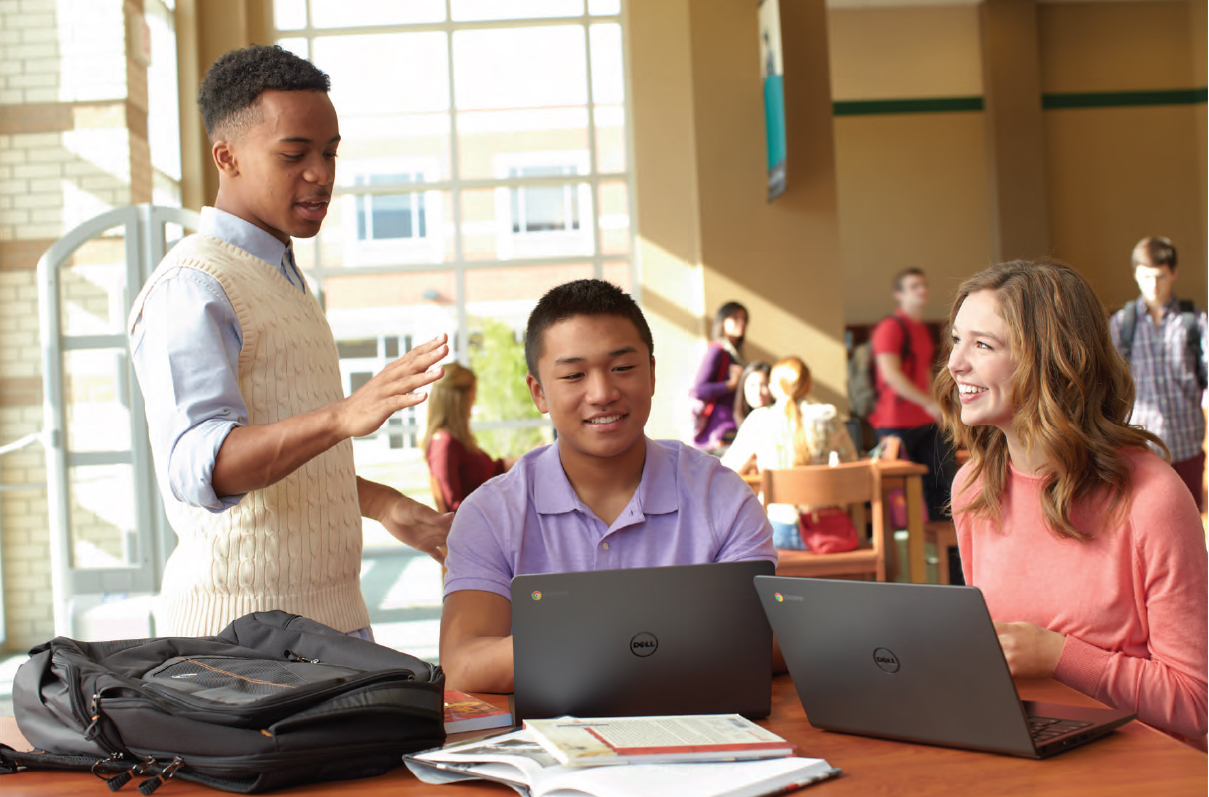The image depicts a bright, sunlit indoor scene in what appears to be a student common area, possibly a library or university student hall. In the foreground, there’s a table cluttered with open textbooks, papers, a black backpack, and two open silver-gray Dell laptops. Two students, who appear to be in their late teens or early 20s, are seated at the table. On the right is a young woman with shoulder-length brown, possibly strawberry blonde hair, wearing an orange or pink sweater, and she is smiling while looking at a man standing nearby. To her left sits a young man of Asian descent in a purple or lavender shirt, attentively looking at his laptop with a smile on his face. 

Standing to the left of the table is an African-American male, engaged in conversation with the seated students. He is characterized by his clean-cut appearance, wearing a white or cream-colored vest over a blue shirt, with his hand raised as if explaining something. In the background, muted and slightly blurred, there are several other students either seated at tables or walking around, and a large window allows sunlight to pour into the room, revealing another building outside. The atmosphere appears to be one of casual study and interaction, blending elements of academia with a relaxed social environment.